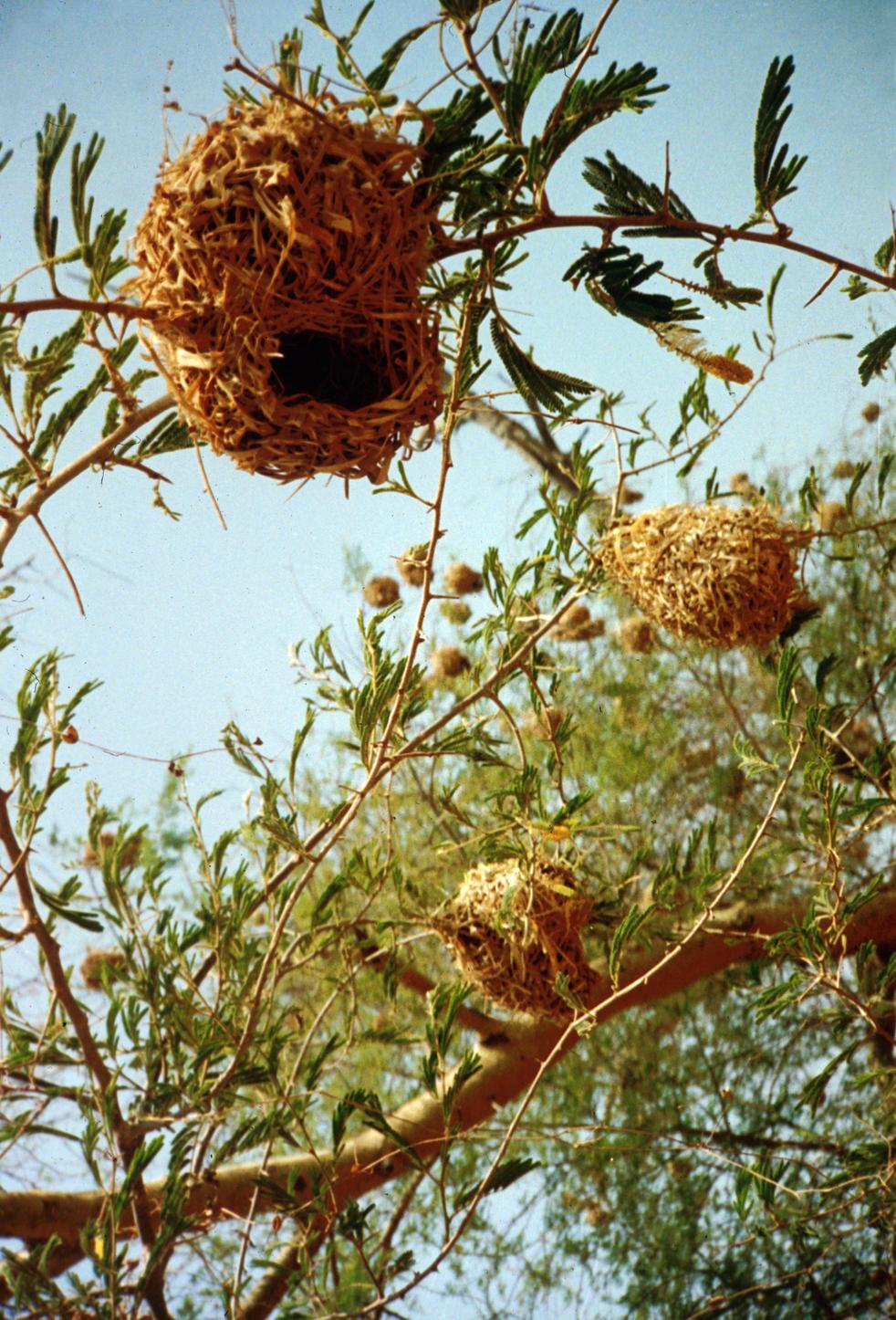The photograph captures a striking scene in nature, taken from an upward angle, looking straight toward the blue sky. It showcases three distinctive bird nests nestled among tree branches and green foliage. The sky in the background is a crisp, light blue, adding to the serene atmosphere of the image.

The main focal points are the nests, uniquely constructed and positioned at different heights on the branches. The largest nest, perched on a higher, smaller branch, is egg-shaped with a woven, straw-like material, featuring a circular entrance at the bottom front. This nest's opening faces the camera lens, revealing a dark interior. The second nest, also on a smaller branch but positioned slightly lower, has a more traditional hemispherical shape, like the bottom half of a ball. The third nest, located on a wider branch towards the bottom of the photograph, appears less complete or not as distinctly shaped but seems to be another traditional nest structure.

This detailed and vibrant photograph beautifully captures the intricacies of the nests amid the lush green leaves and emphasizes the serene blend of natural elements under a sunny, blue sky.